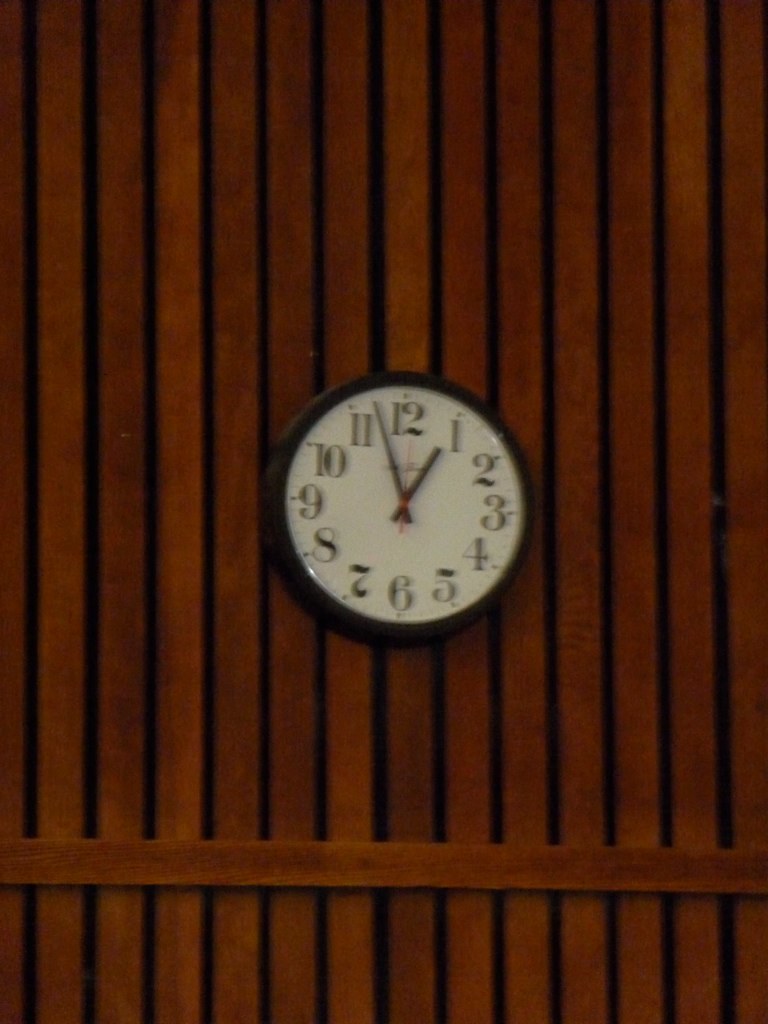The image depicts a traditional, round wall clock with a black circular frame and a stark white face. The clock features large black numbers from 1 to 12 and minute markers around the circumference. The hour and minute hands are black, while the second hand is red. The clock is set at approximately 12:55, with the hour hand near the 1 and the minute hand between the 11 and 12. The background consists of vertically aligned wooden planks with a cherry wood finish, exhibiting small gaps between them. A horizontal plank intersects these vertical panels near the bottom of the image. The photograph appears slightly blurry, adding a subtle out-of-focus effect to the overall composition.